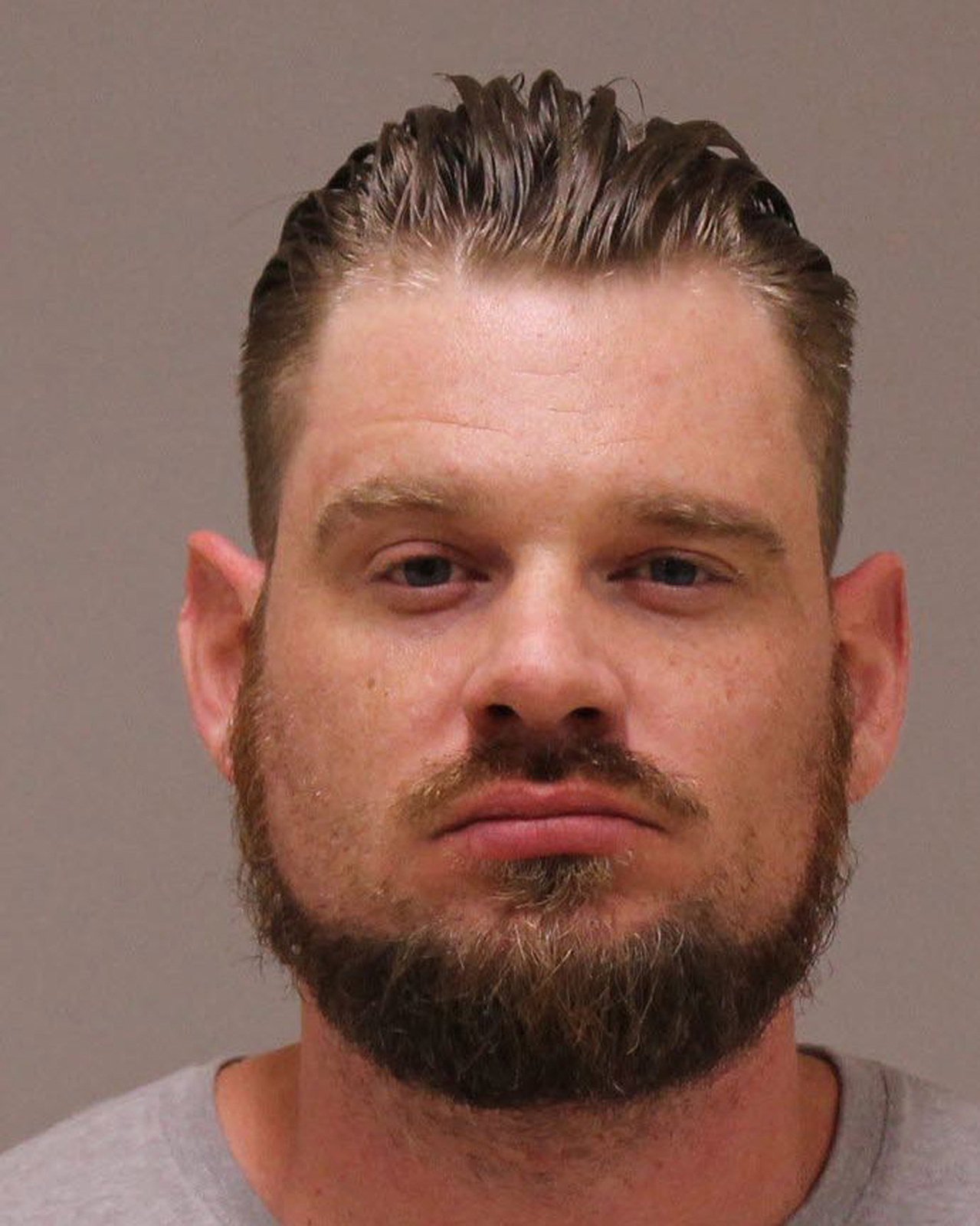In this detailed, full-color photograph, a Caucasian man with an intense, slightly grimacing expression stands against a vertically rectangular, gray background. The artificial light creates a gradient, darker at the top and lighter towards the bottom. He has short, greased-back brown hair without a part and pointy ears that stick out slightly. His face features include light-colored eyes, brown eyebrows with a blondish tint, and visible forehead wrinkles. His pink lips are closed, adding to the serious look on his face.

The man sports a full, scraggly beard that extends up to his hairline, resembling sideburns merging into a fuller beard, but it also includes long and untidy neck hair. He has a mustache, and his neck shows signs of stubble beneath a white, shaved area. He is dressed in a gray T-shirt, which gets cut off at the bottom of the image. The background behind him is a brownish-gray color, contributing to the overall simplicity of the photograph. The focus remains on his face, taking up the central portion of the frame, suggesting this might be a portrait or a photo shoot lineup.